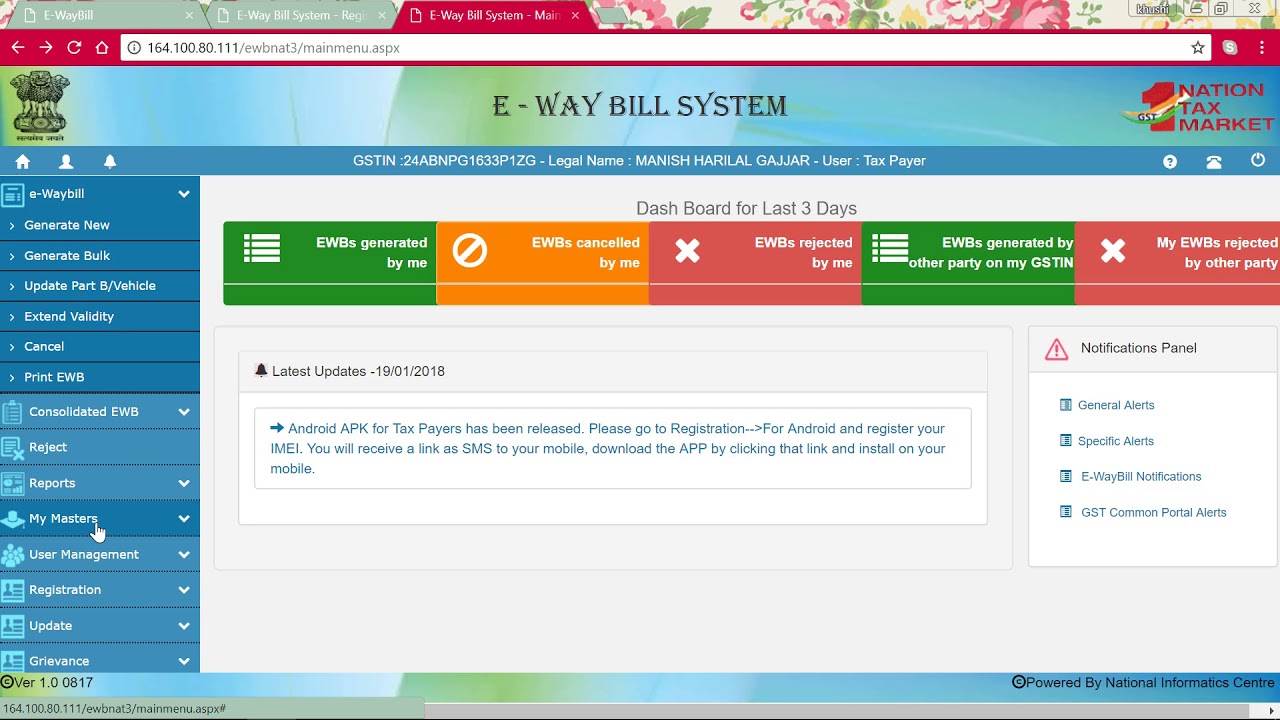This image is a detailed screenshot of a website displayed on someone's computer. The URL in the address bar reads "EWB NAT 3/mainmenu.aspx." At the top left of the page, within a small rectangular box with a blue and green gradient background, the text "E-Way Bill System" is prominently featured in black. Adjacent to this, in red text, the site reads "National Tax Market" followed by the number 1.

Below this header, a blue rectangular section contains various details, including the legal name "Manish Haril Gajjar." Further down, a section titled "Dashboard for last three days" is visible, displaying a row of five colored rectangles. These rectangles come in distinct colors—green, orange, and pink—and each represents different statuses: "Generated by Me," "Canceled by Me," "Rejected by Me," "Generated by Other Party on My GSTIN," and "Rejected by Other Party."

Below the dashboard section is a part labeled "Latest Updates," which provides additional information. To the right of this, the "Notifications Panel" is displayed, with categories listed in blue such as "General Alerts," "Specific Alerts," "E-Way Bill Notifications," and "GST Common Portal Error Alerts."

On the far left side of the screenshot, there is a vertical menu consisting of several little blue rectangles with white text, each representing different navigational options for the website.